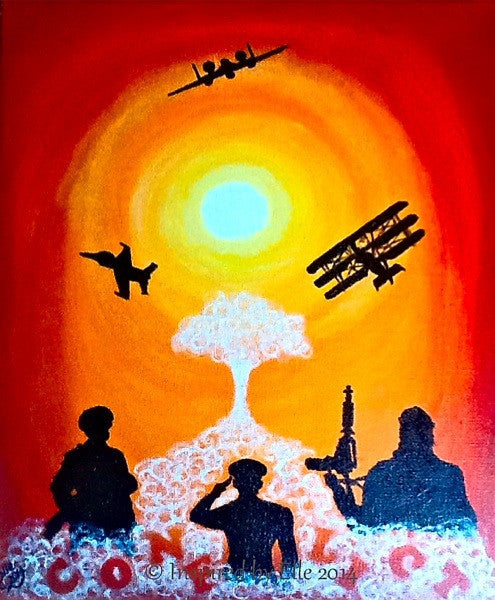The painting depicts a highly stylized and symbolic scene with silhouetted characters set against a bold, concentric color gradient. At the center top of the frame is a bright yellow sphere that resembles a sun, surrounded by circles of color transitioning from yellow to orange, and eventually to dark red at the edges, creating an arch-like shape. Silhouetted across this vibrant backdrop are three aircraft: a modern fighter plane head-on at the top, an old-fashioned triple-winged plane facing away in the bottom right, and an angled modern jet fighter to the left of it. Dominating the center bottom is a mushroom cloud formed by a pile of white circles, with three soldiers in varying stances silhouetted against it. The soldier on the left dons a beret, the middle soldier salutes while wearing a cap, and the rightmost soldier holds an assault rifle pointed upward. Below these figures, interspersed among the white circles, the word "CONFLICT" is displayed in striking red text. The overall mood and elements of the painting suggest a contemplation of historical and modern warfare.